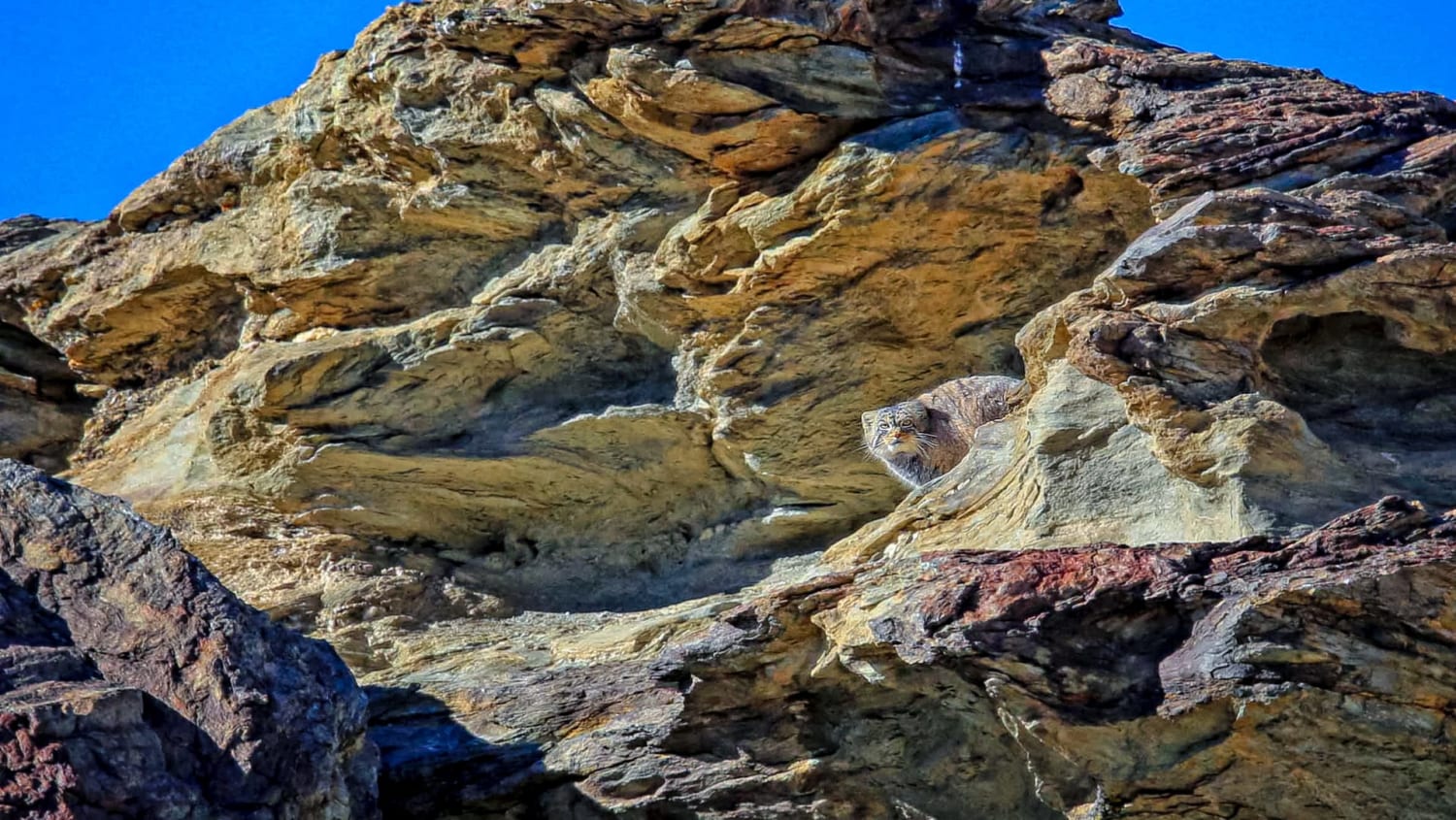The image showcases a vast, mountainous region dominated by an expanse of rocky terrain. The scene is characterized by layers upon layers of rocks that ascend steeply, creating a seemingly endless rocky expanse. The rocks vary in colors, with dark browns and grays in the foreground, transitioning to lighter grays, reds, whites, and even hints of golden hues, possibly reflecting sunlight. The vastness of the rocky landscape is set against a backdrop of a partly cloudy, blue sky, visible at the edges of the photo. 

Amidst the rocks on the mid-right of the image, a camouflaged Bobcat blends seamlessly with the rocky environment, peering down towards the camera. This adds a subtle touch of life to the otherwise barren, rugged scene. The terrain appears extremely jagged and complex, with no visible ground other than rock formations, giving an impression of a desolate, desert-like area. Shadows add depth to the rocky layers, emphasizing the height and various levels of this imposing rocky cliff.